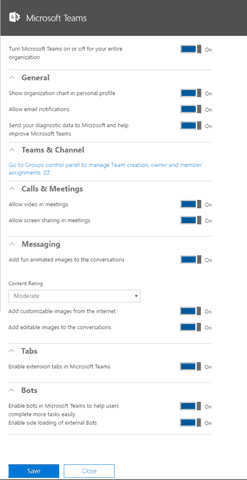The image shows the settings page within the Microsoft Teams application on a smartphone. At the top, there is a header bar displaying "Microsoft Teams." Below the header is an extensive list of settings categories, each accompanied by a toggle switch designed to enable or disable specific options. 

The settings categories include:
1. **General Settings**
2. **Teams and Channels**
   - Accompanied by blue hyperlink text for additional options (text content is not legible).

3. **Calls and Meetings**
   - Contains two sub-settings.

4. **Messaging**
   - Features one standalone setting and another with a dropdown menu, followed by two additional settings.

5. **Tabs**

6. **Bots**

At the bottom of the settings page, there are options to "Save and Close" or "Cancel" any changes made. The layout indicates a user-friendly and intuitive interface designed for easy navigation and customization of personal preferences in Microsoft Teams.